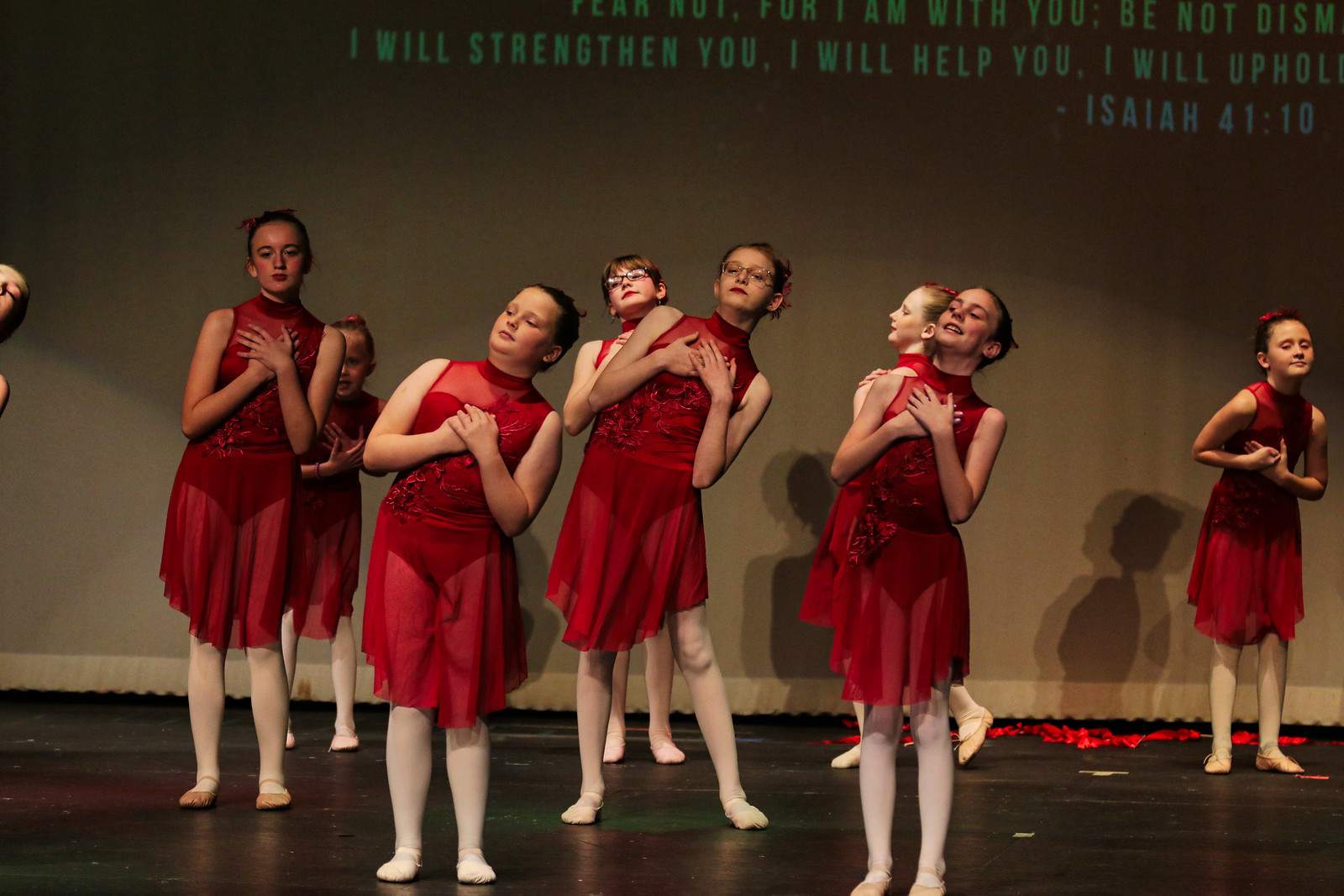This is a color photograph capturing an indoor scene featuring nine young girls performing on a wooden stage stained a dark color. The girls are dressed in deep red, sleeveless ballet costumes with white stockings and ballet shoes, exuding a polished and graceful appearance. Scattered red leaves adorn the stage, adding a touch of whimsy to the scene. 

In the midst of their performance, the girls are positioned with both hands clasped to the middle of their chests, appearing to lean slightly to the side. Some of them have their eyes closed, and they exhibit varied expressions, suggesting an emotional connection to their act. 

Behind them is a large curtain partially obscuring text from a Bible verse, Isaiah 41:10-17, displayed on a projector screen. The visible portions read, "Fear not, for I am with you; be not dismayed... I will strengthen you, I will help you, I will uphold..." The photograph cuts off parts of the verse. This evocative image captures a poignant moment in the girls' performance, set against a backdrop of faith and empowerment.